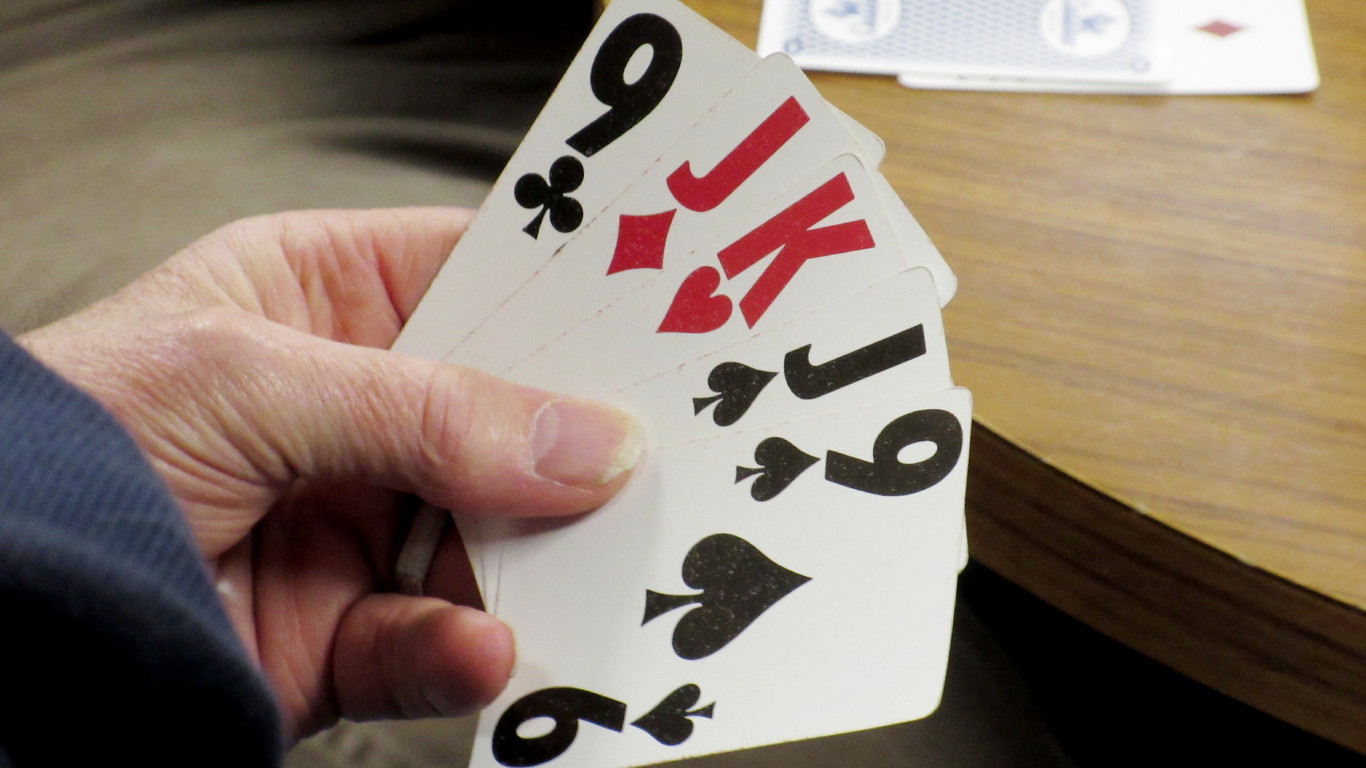The image features a close-up view of a hand holding a fanned arrangement of playing cards over a wooden table. The table has a distinct round, curved edge, showcasing a light brown surface with visible dark brown grain lines. On the table are two additional cards: one placed face up revealing a diamond, and the other face down, its identity hidden. The hand in the image appears unmanicured and displays five cards spread out like a fan. The cards include a nine of clubs, a jack of diamonds, a king of hearts, a queen of spades, and a nine of spades.